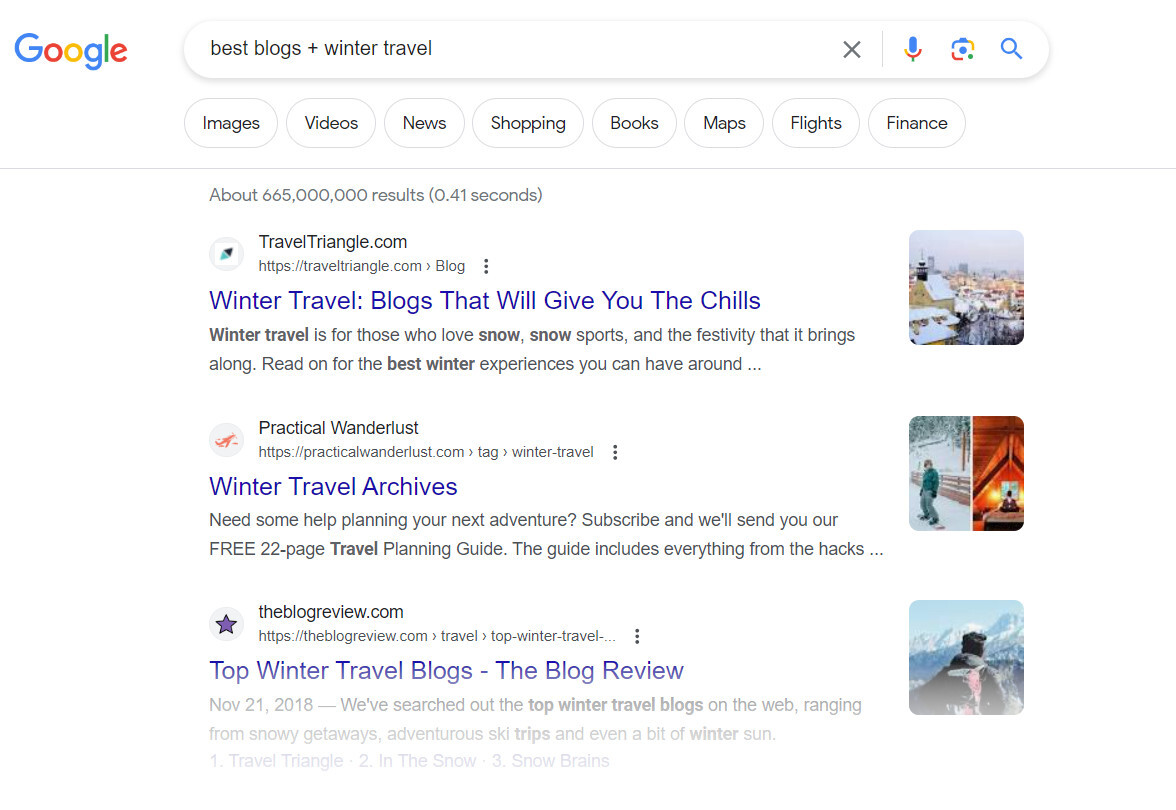A screenshot of a Google search results page for "best blogs winter travel." The browser interface displays various filtering options, such as Images, Videos, News, Shopping, Books, Map, Flights, and Finance. The first search result is from TravelTriangle.com, with the title "Winter Travel Blogs That Will Give You the Chills" accompanied by a small thumbnail image. The second result is from Practical Wanderlust, labeled "Winter Travel Archives," also featuring a thumbnail image. The third result comes from TheBlogReview.com, titled "Top Winter Travel Blogs – The Blog Review," with an additional thumbnail. The search result titles are prominently presented in purple text, while the additional information appears in gray text. Thumbnail images associated with the results exhibit scenic winter landscapes: cities covered in snow, a person snowboarding down a snowy hill, an A-framed cabin with a cozy fire visible inside where someone is relaxing on a bed, and an individual standing before a majestic snowy mountain.